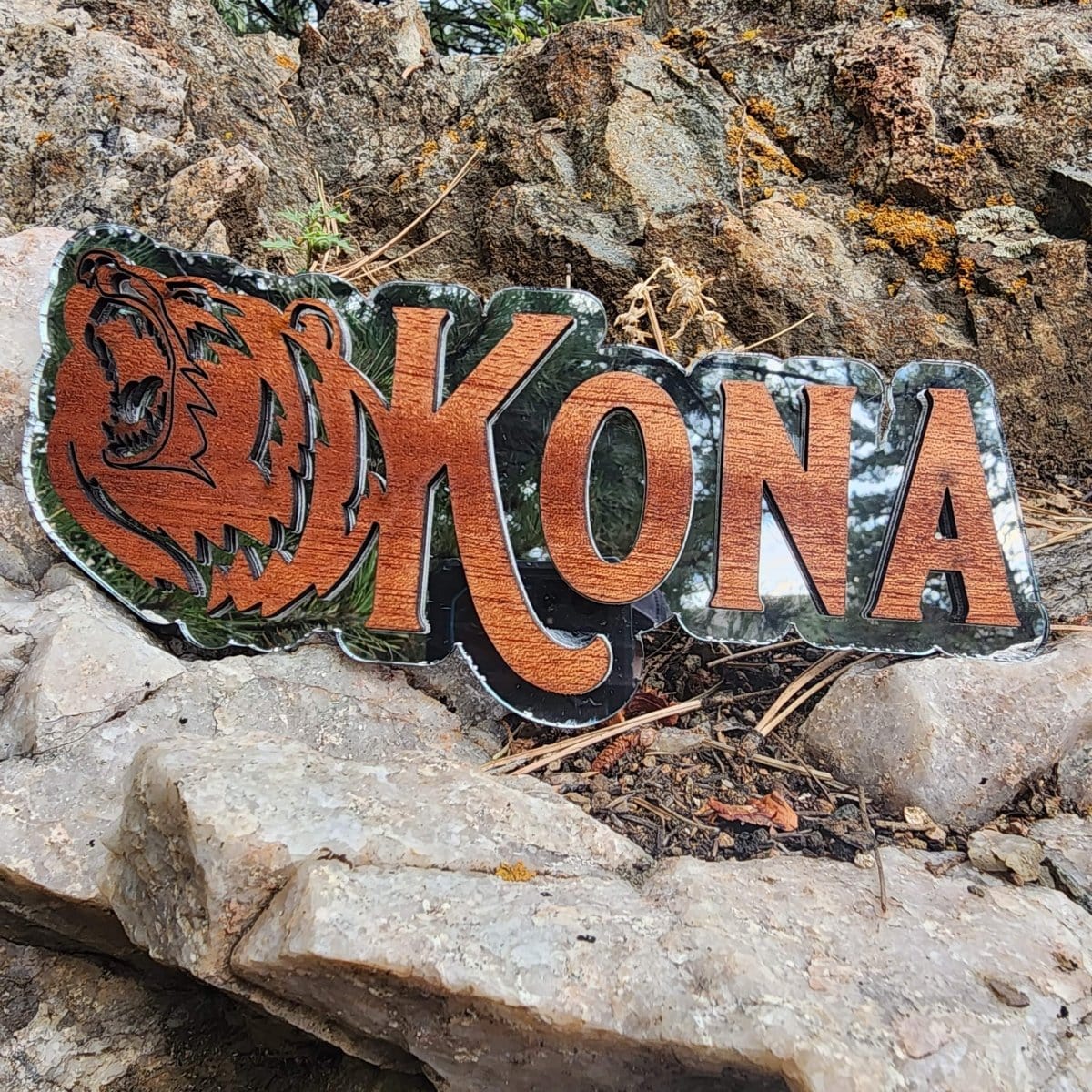The photograph captures a rugged, outdoor scene dominated by a rocky hillside. The bottom of the image showcases large, light-colored rocks interspersed with twigs, dried grass, and small stones; there is even a noticeable gap under one of the rocks in the lower left-hand corner. Ascending the hillside, you notice the rocky landscape continues, adorned with patches of orange moss and sparse grass sprouting up, particularly in the upper sections. Centered in this natural setting is a striking wooden sign with the word "Kona" engraved on it. The letters are cut out against a carved depiction of a roaring bear to the left. This sign rests on a small rocky ledge, distinct from the surrounding hill. The background behind the sign is reflective, hinting that the board might be made of glass, capturing subtle reflections of nearby trees.